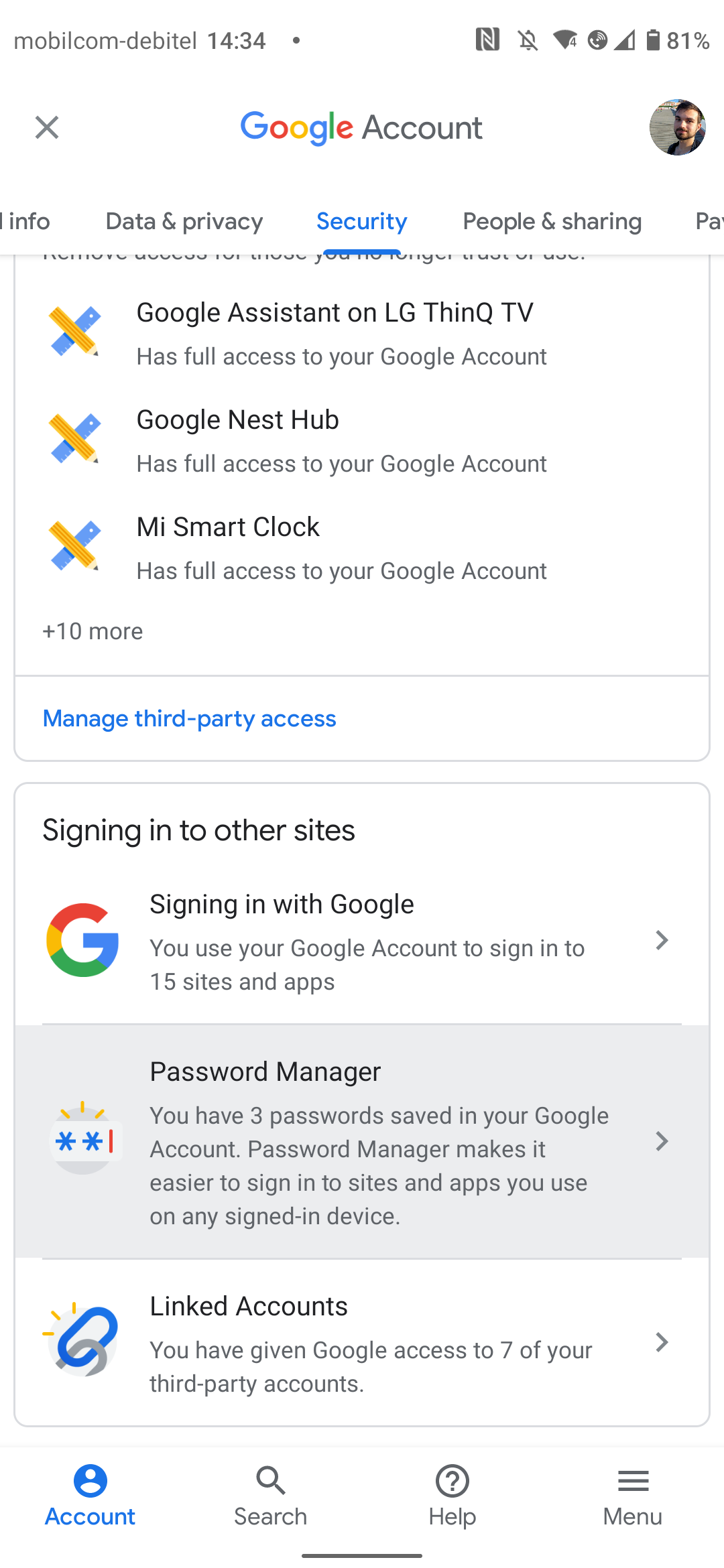This image is a screenshot of a Google account page taken from a smartphone, as indicated by the status bar in the top right corner showing the battery level at 81%. The time displayed in the top left corner reads 14:34, reflecting military time.

The page being viewed is the "Security" section of the Google account settings. The background of the page is white, contrasting with the black text. Key sections visible on the screen include "Signing in with Google," "Password Manager," and "Linked Accounts." 

Near the bottom of the screenshot, there are four options: a light blue button labeled "Account" positioned on the bottom left, and three icons to the right for "Search," "Help," and a menu option. 

In the top right corner of the page, the profile picture of the account holder, who appears to be a male, is visible. Centrally placed at the top of the page, the title "Google Account" is displayed in bold. This detailed screenshot effectively captures the important elements of the Google account's security settings interface.